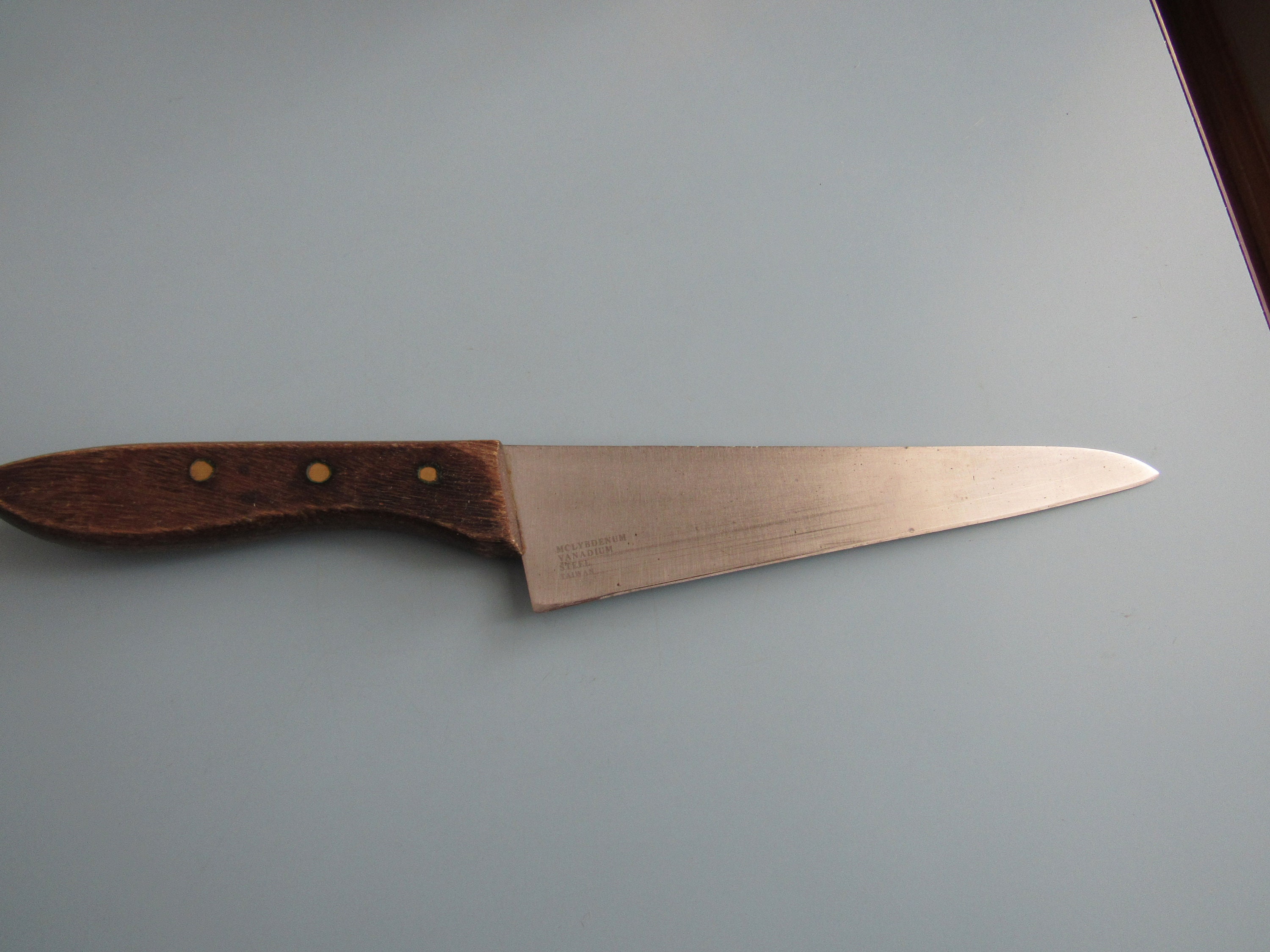A steak knife sits on a light gray kitchen counter. The blade is wide at the base and narrows to a pointed tip, with an upper edge that rounds slightly before leveling off straight back. The silver-gray steel displays horizontal scratches following the cutting edge, indicating signs of wear and age, with areas even starting to brown. The handle, made of worn dark brown wood, curves at the bottom to fit comfortably in the hand and features three orange-colored, slightly worn rivets. The handle shows heavy use, with visible hand oils fading its edges. In the upper right corner of the image, a black triangle can be seen, contrasting with the shadowy, gray-toned surface of the countertop.